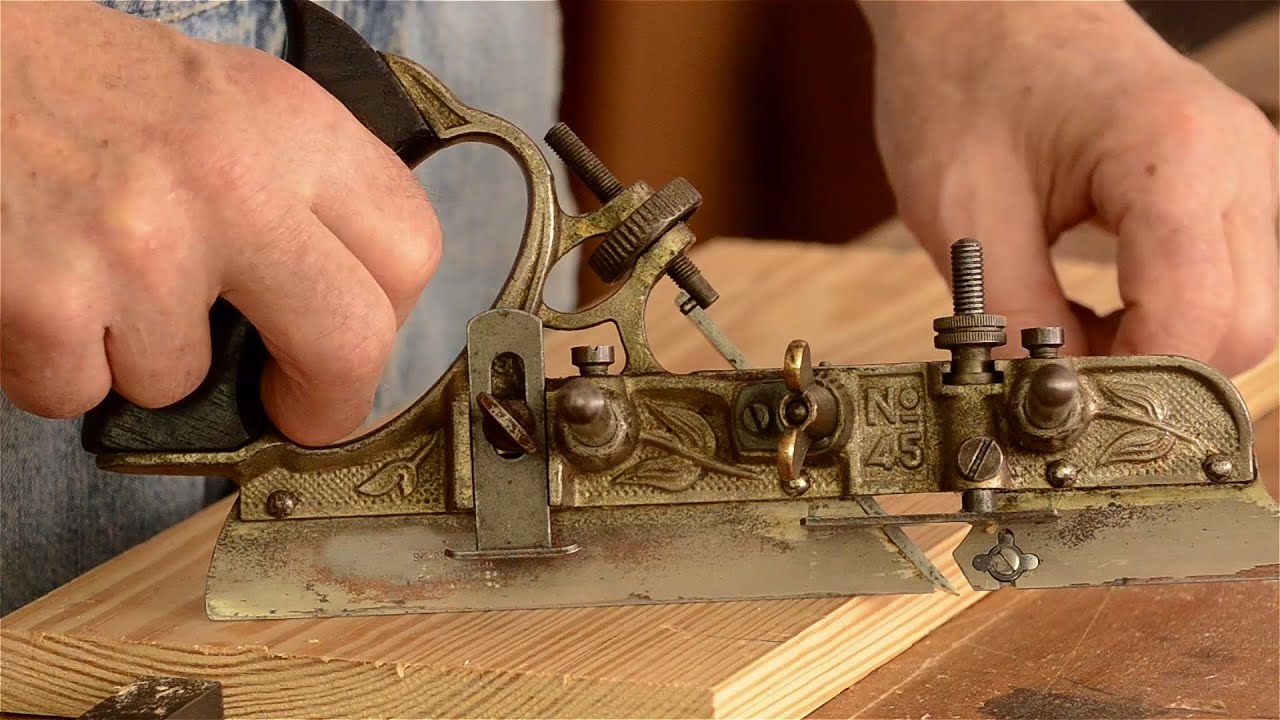This photograph, taken indoors, captures a close-up of a person using an old combination plane on a wooden board, which rests on a wooden workbench. The focal point of the image is the vintage combination plane, identified as a No. 45. It features intricate floral or leaf designs on its center and is constructed from brass, with visible signs of discoloration and rust. The tool includes a large, candle-shaped handle on the back, gripped by the person's right hand. Notably, there are screws, gears, and adjustable levers integrated into its design, including a prominent wing nut in the center resembling a propeller. The plane has two blades beneath it— a larger back blade and a smaller front blade, making it effective for shaving and polishing wood. The person's left hand is holding down the wooden board, which appears natural and unpolished. The manual effort involved in using this antique tool is evident, emphasizing the craftsmanship and care of traditional woodworking methods.